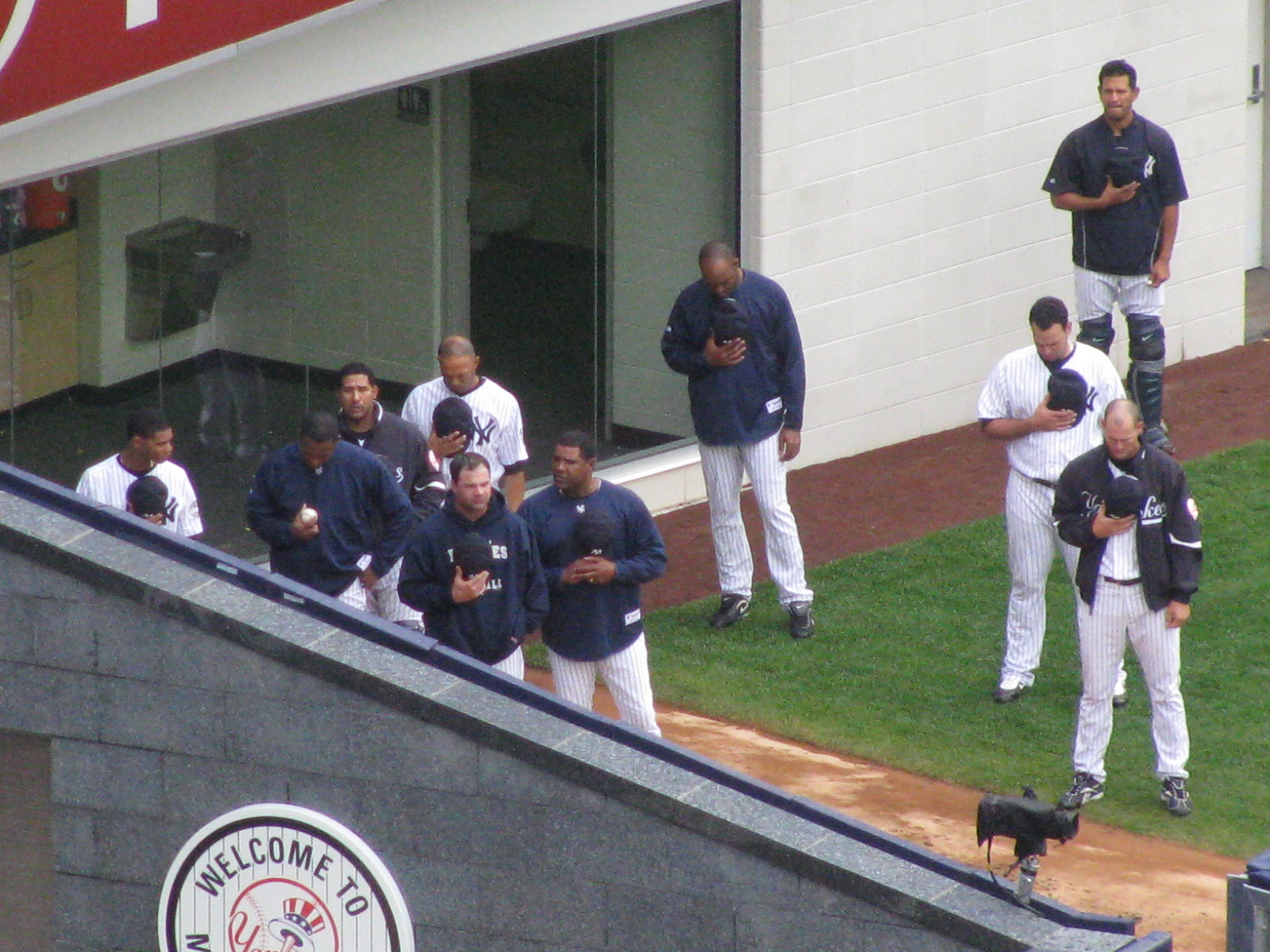The image captures a detailed top-down view of the warm-up area at a baseball stadium. In the corner of this area, approximately ten New York Yankees players are positioned near a building with a glass front. Through the glass, a bathroom with a unisex sign and a water fountain are visible. The floor inside is dark gray, and the building itself is constructed of white concrete blocks. At the top of the building, a red banner with white writing is prominently displayed. The players, dressed in distinctive Yankees uniforms featuring white with light blue pinstripes, are standing solemnly with their hats removed and held against their chests, likely reciting the Pledge of Allegiance or the national anthem. Some players are also wearing navy blue long-sleeve shirts or windbreaker jackets. In the bottom left corner of the image, there are gray concrete blocks with a partially visible emblem reading "Welcome to" with the "N" for New York and part of the Yankees logo.